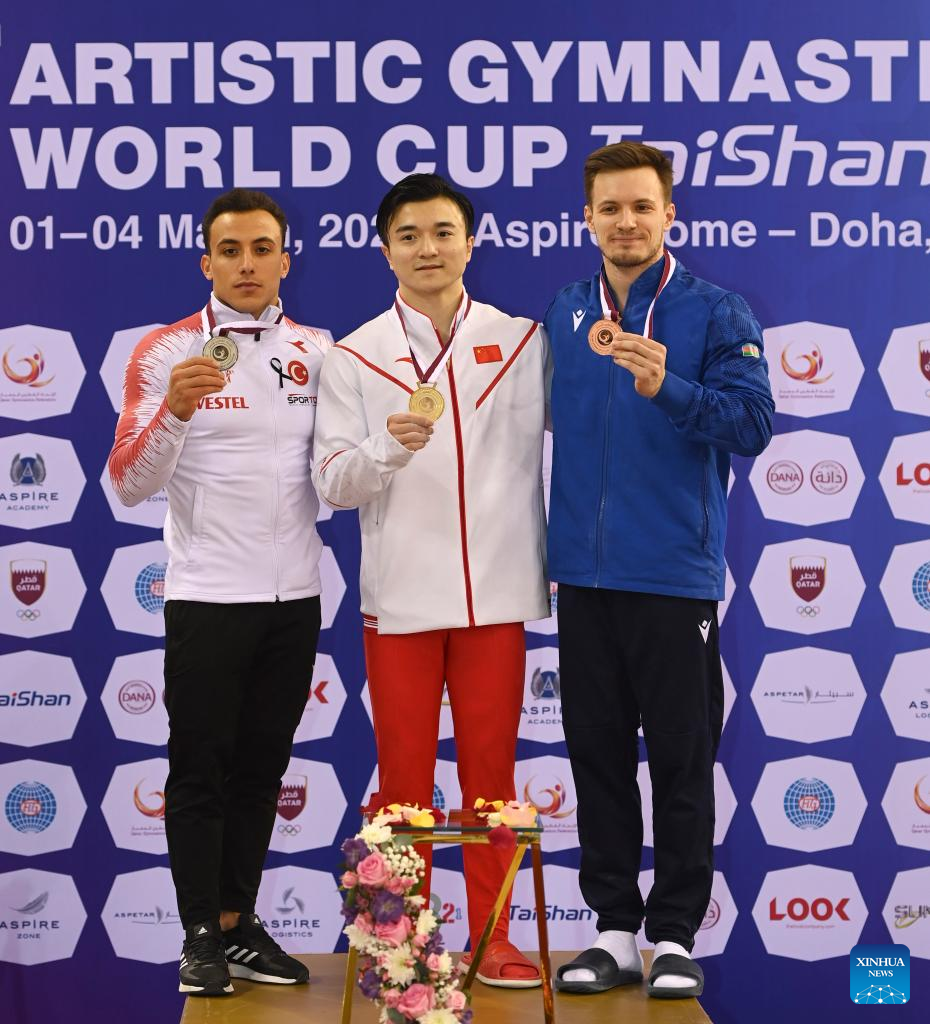The photograph captures a significant moment at the Artistic Gymnastics World Cup, showcasing three medalists standing triumphantly on a podium. The background is a rich blue adorned with various sponsor logos and a prominent white text header reading "Artistic Gymnastics World Cup," partially obscured by the athletes' heads. 

In the center stands the gold medalist of Asian descent, wearing a white jacket with the Korean flag and red pants, proudly holding his gold medal aloft. To his left, the silver medalist, who appears to have dark features possibly of Mexican descent, dons black track pants and a white jacket with orange flame-like patterns down the sleeves, displaying his medal. On the right, the bronze medalist, a man with brown hair and white complexion, wears black track pants and a blue tracksuit top, also holding his medal.

At the base of the podium, a wooden stand with a floral arrangement adds a touch of elegance to the celebratory scene, complemented by additional floral pieces. In the bottom right corner of the backdrop, the logo of XINHUA News is visible, set against a light blue background. The overall image exudes a sense of pride and accomplishment, highlighted by the vivid details of the athletes' attire and the carefully curated background.